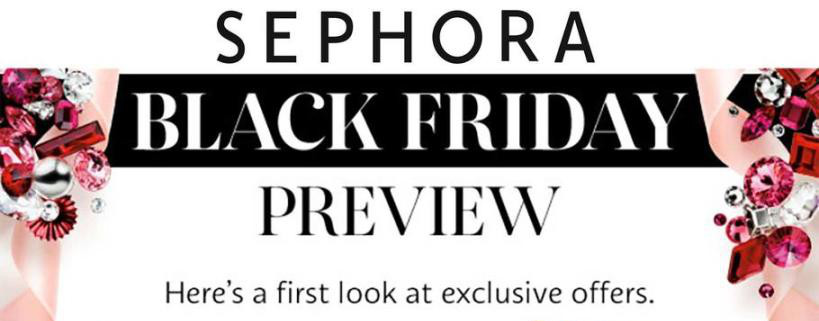The webpage opens with a prominent banner featuring the Sephora logo in sleek black lettering against a clean white background. Just below this, a striking black banner spans the width of the page, displaying "BLACK FRIDAY" in bold, all-caps white letters. Beneath this eye-catching announcement, the word "PREVIEW" is showcased in black letters on a white background, offering a preview of upcoming deals. While the fonts for "Sephora," "Black Friday," and "Preview" differ, "Black Friday" and "Preview" share a similar style, though the latter is not bolded.

Flanking this central information, festive colors of red, silver, and black adorn the sides, set against a seemingly pink cloth, evoking a seasonal, Christmas-related theme. At the bottom of the banner, text reads: "Here's a first look at exclusive offers," inviting visitors to get a sneak peek at special Black Friday deals and potentially save money on their holiday shopping extravaganza.